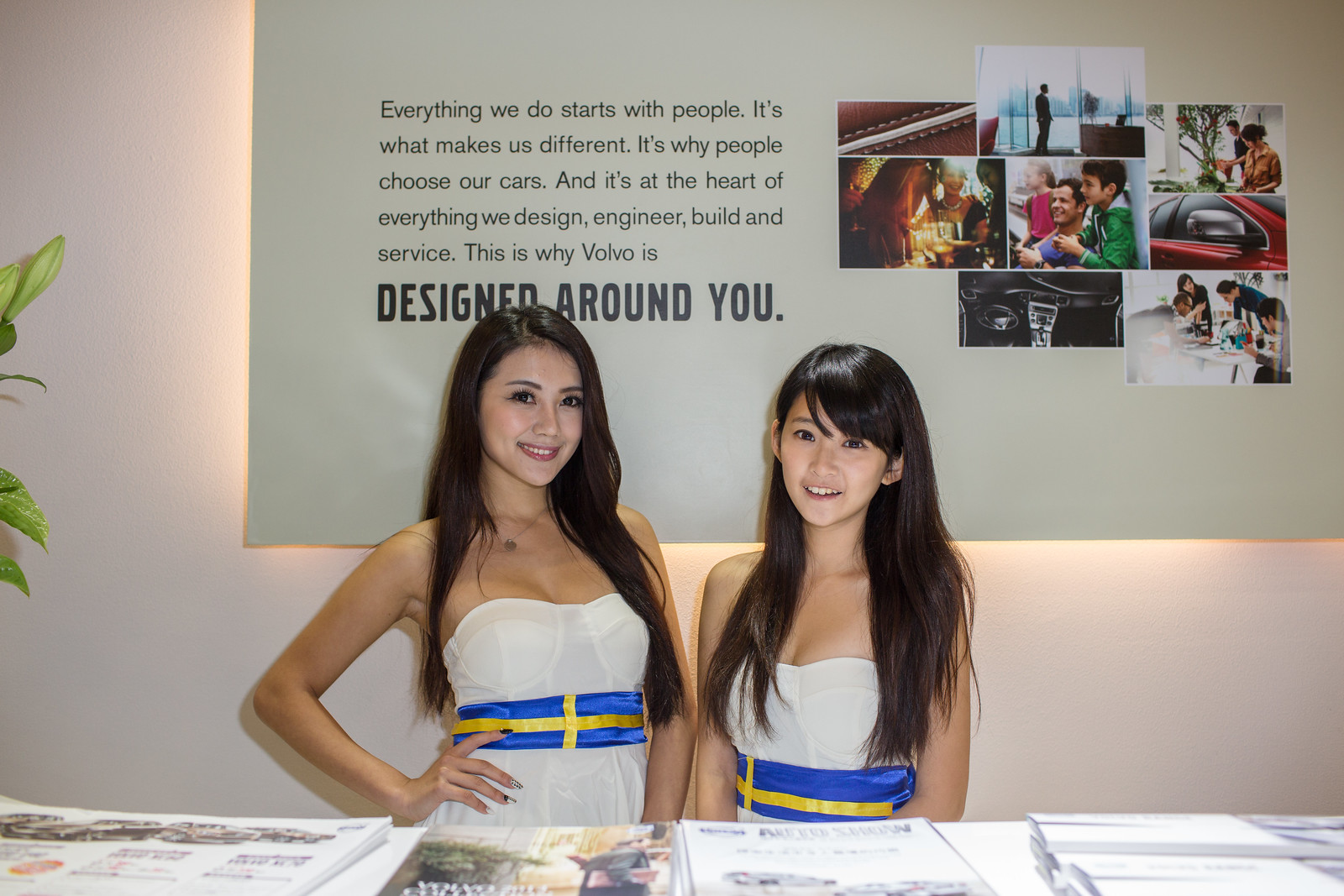In the wide rectangular image, two smiling women, both with light Asian skin and long brown hair, pose in front of a light green sign. They are wearing strapless white dresses accentuated with sashes that are bright blue and feature a gold cross. The background is an off-white wall, and at the bottom of the image, a white table surface is covered with various magazines and flyers. Above the women, the prominent sign reads in black font: "Everything we do starts with people. It's what makes us different. It's why people choose our cars. And it's at the heart of everything we design, engineer, build, and service. This is why Volvo is designed around you." The sign also includes several pictures on the right, presumably of Volvo customers.